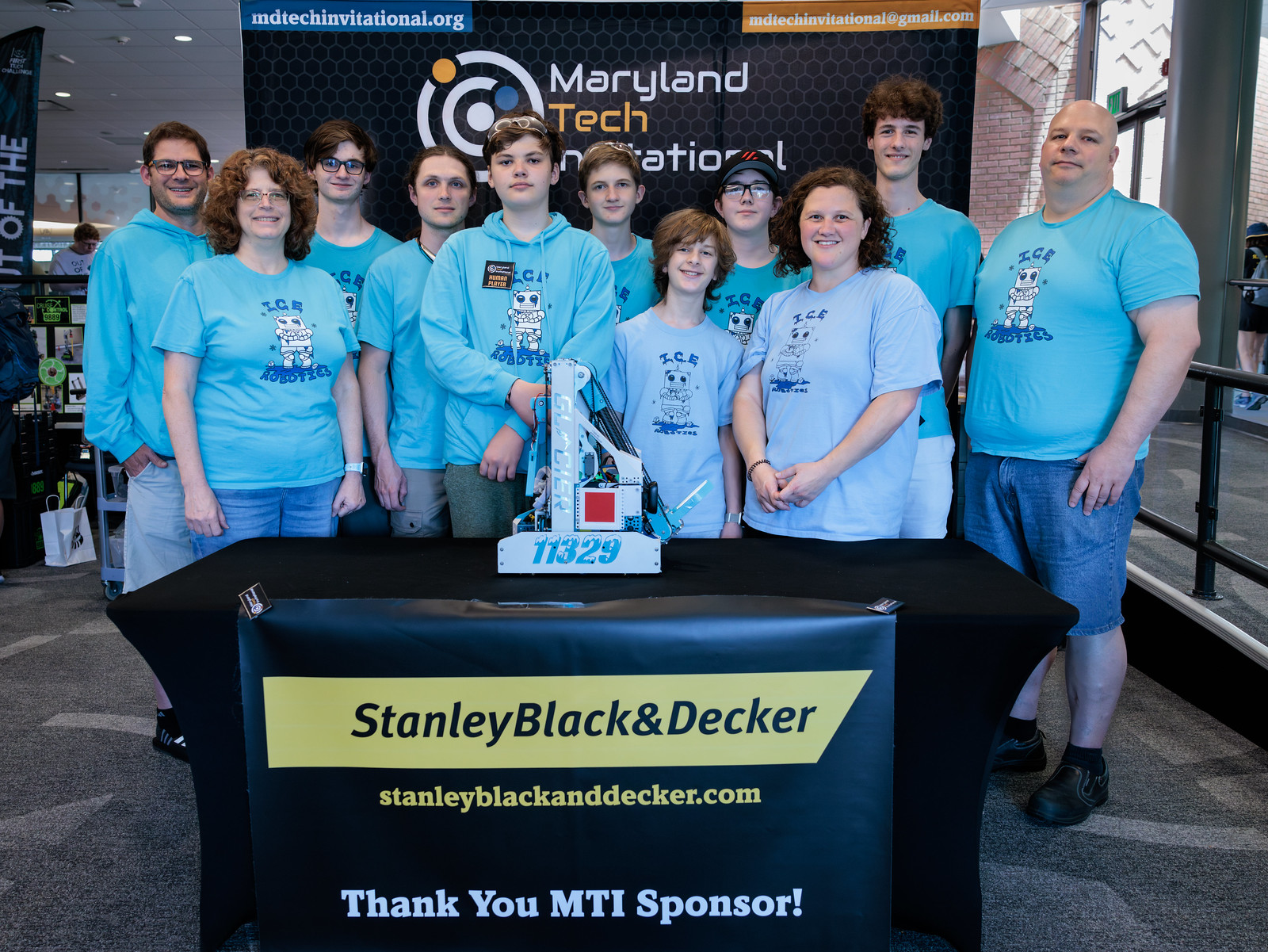This image captures a diverse group of approximately ten individuals, both men and women of varying ages and sizes, standing behind a counter. Each person is clad in a turquoise shirt or sweatshirt emblazoned with a white robot graphic and text above and below the image that reads "ICE Robotics." The backdrop behind them is a black wall with the text "Maryland Tech International," accented with concentric white circles and colors such as blue and orange, suggesting a tech-oriented backdrop likely related to a tech convention.

The counter they stand behind is draped with a black banner proclaiming "Stanley Black & Decker" alongside the sponsor's URL, stanleyblackanddecker.com. This banner also contains the text "Thank you MTI sponsor" in white and gold lettering. Additionally, there appears to be some sort of contraption on top of the counter with the number 11329, possibly showcasing a project by the team. A blue, white, and red design is visible atop the displayed table, highlighting the team's creative efforts. The overall scene suggests a formal group photo taken during a tech event, where the team is proudly presenting their work.